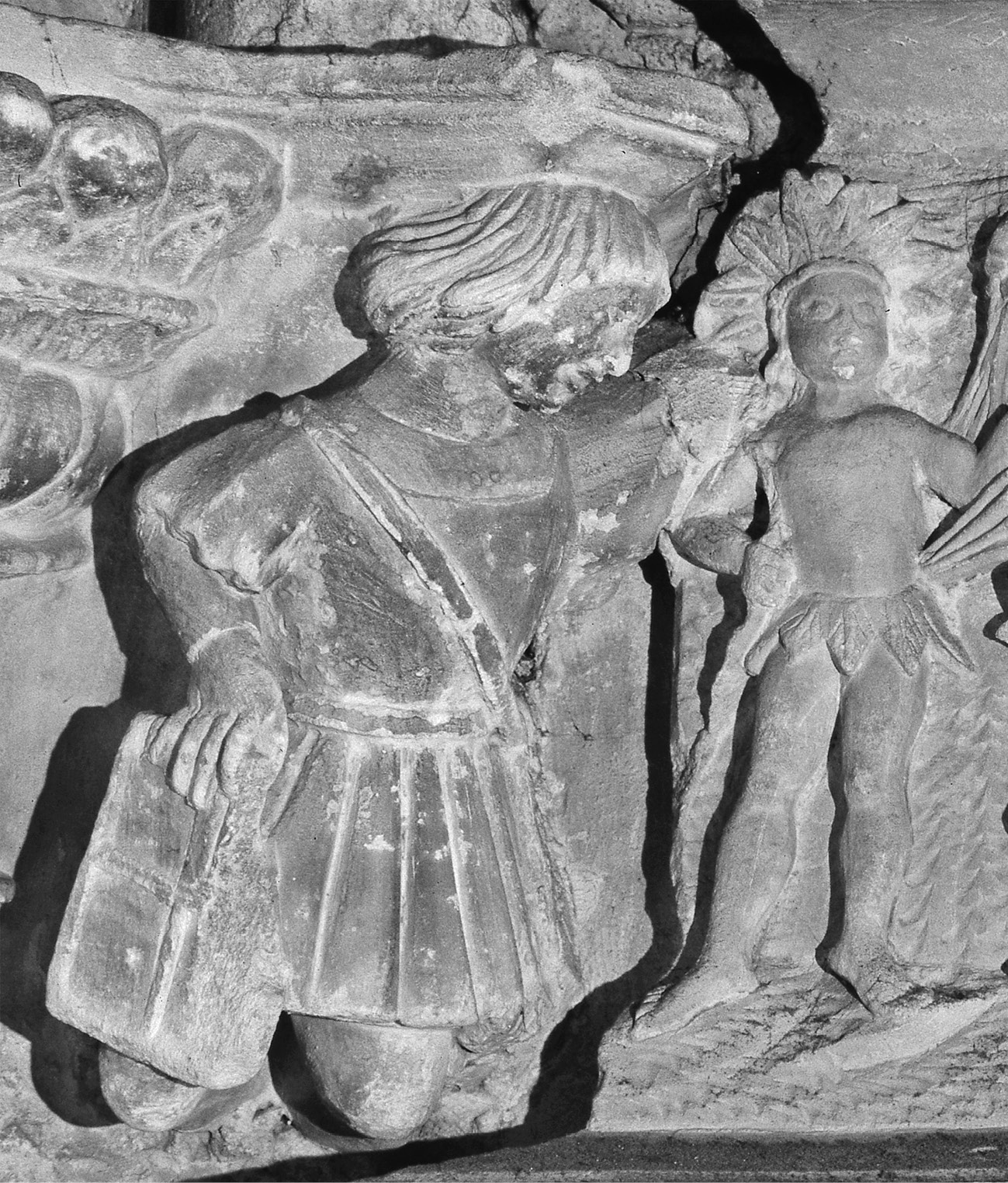The black and white photograph captures the intricately carved stone artifacts that appear to be part of ancient ruins, possibly found in a cave and taken with night vision. The scenes depict two figures: a man with shoulder-length hair wearing a pleated skirt and holding a tablet in his left hand. He is kneeling next to a small child standing to his right. The child is adorned in a leaf skirt and headdress, standing barefoot with hands on his hips, looking outward. The carvings show considerable age, with pieces broken off, and the stone appears dark, worn, and distressed, enhancing the sense of antiquity and historical significance.